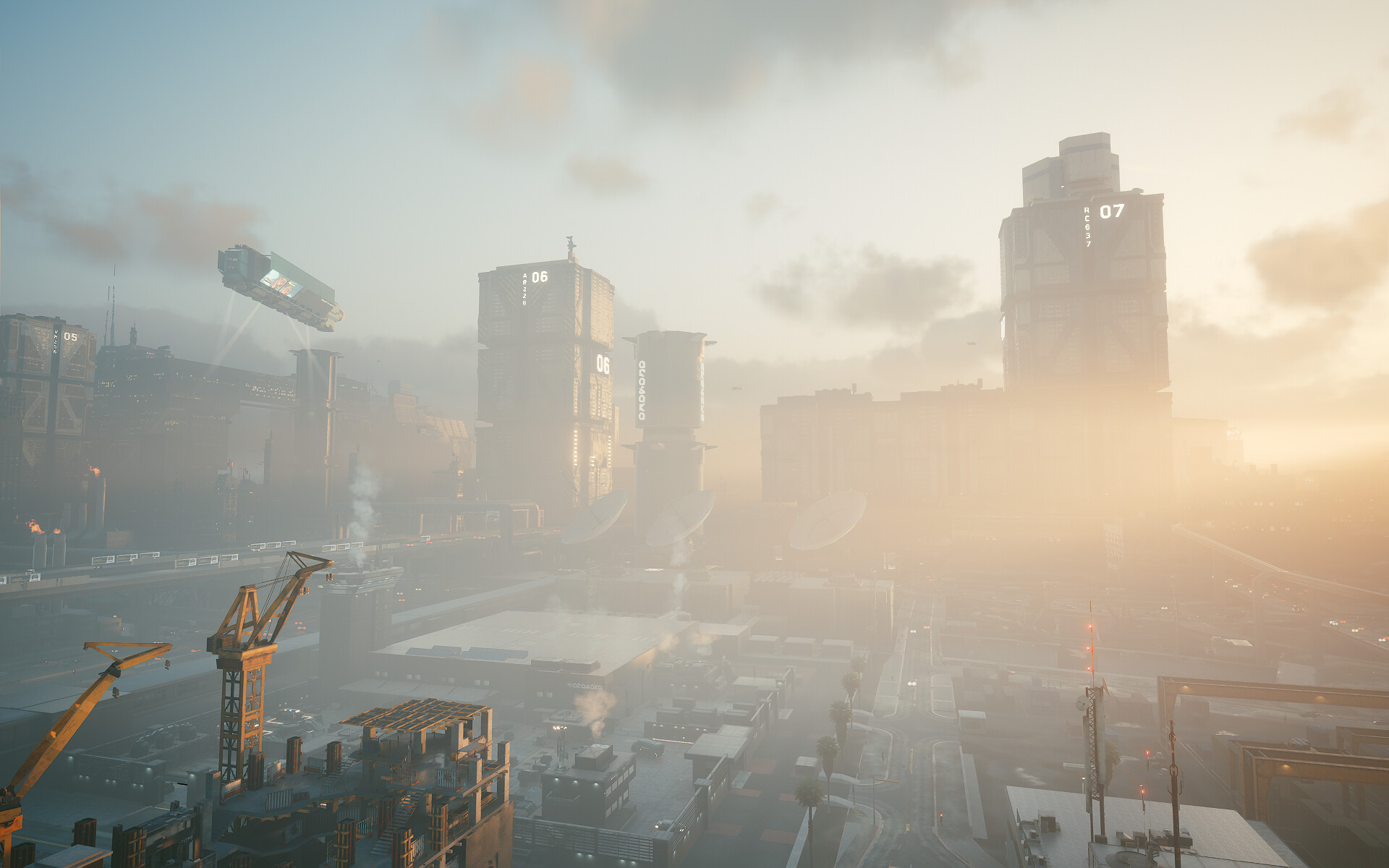The image presents a surreal, sci-fi-inspired industrial cityscape shrouded in a light fog. Central to the scene are two buildings prominently numbered with fluorescent '06' and '07'. Morning sunlight glows through the haze, casting an eerie ambiance across the area. On the left side of the picture, a unique airship—resembling a blimp but shaped like a long cylindrical octagon—hovers above a building. Lights from this airship illuminate the structure below, suggesting it may be tethered for surveillance or transportation purposes.

In the foreground, an array of cranes points to ongoing construction activities, adding to the industrious atmosphere. The environment is punctuated with red aircraft warning lights, contributing to the scene's otherworldly feel. The sky above is a gradient of dark blue fading into a brighter blue towards the right, where the sun rises, painting the horizon with a warm orange hue. Wisps of puffy clouds are visible through the mist, enhancing the ethereal quality of this futuristic tableau.